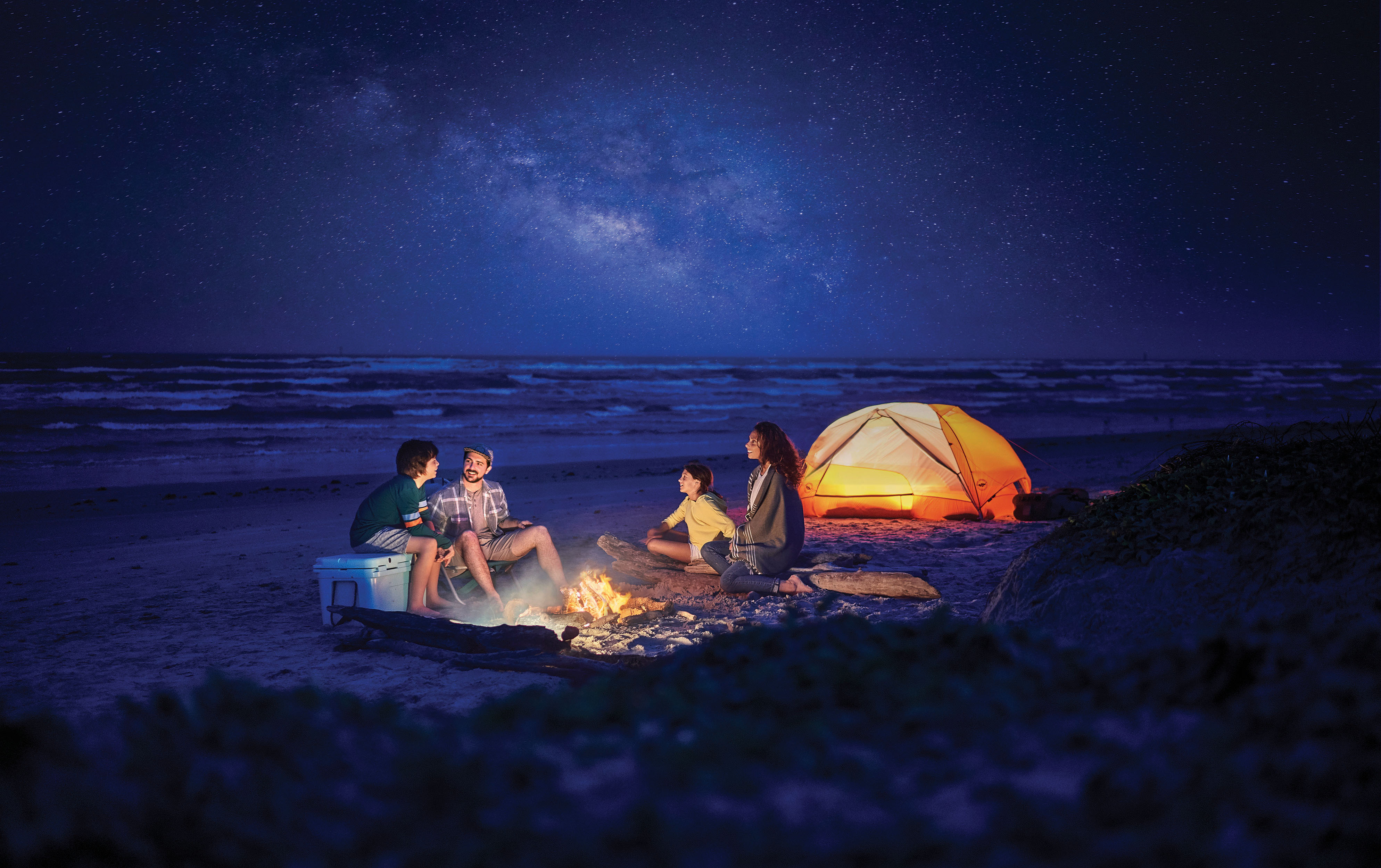A serene nighttime scene at the beach features a family camping setup by the ocean. A warmly lit tent is pitched in the sand, casting a welcoming glow in the soft purple hues that pervade the entire scene. The mother, father, and their children are seated around a small campfire that crackles gently, providing both warmth and light. Beside them, a cooler suggests they have plenty of refreshments for their cozy night under the stars. The sky, ocean, and beach all share a dreamy, violet tint, giving the whole image a magical and tranquil atmosphere. This horizontal photograph captures the family’s intimate moment amidst the natural beauty of the purple-tinted night.